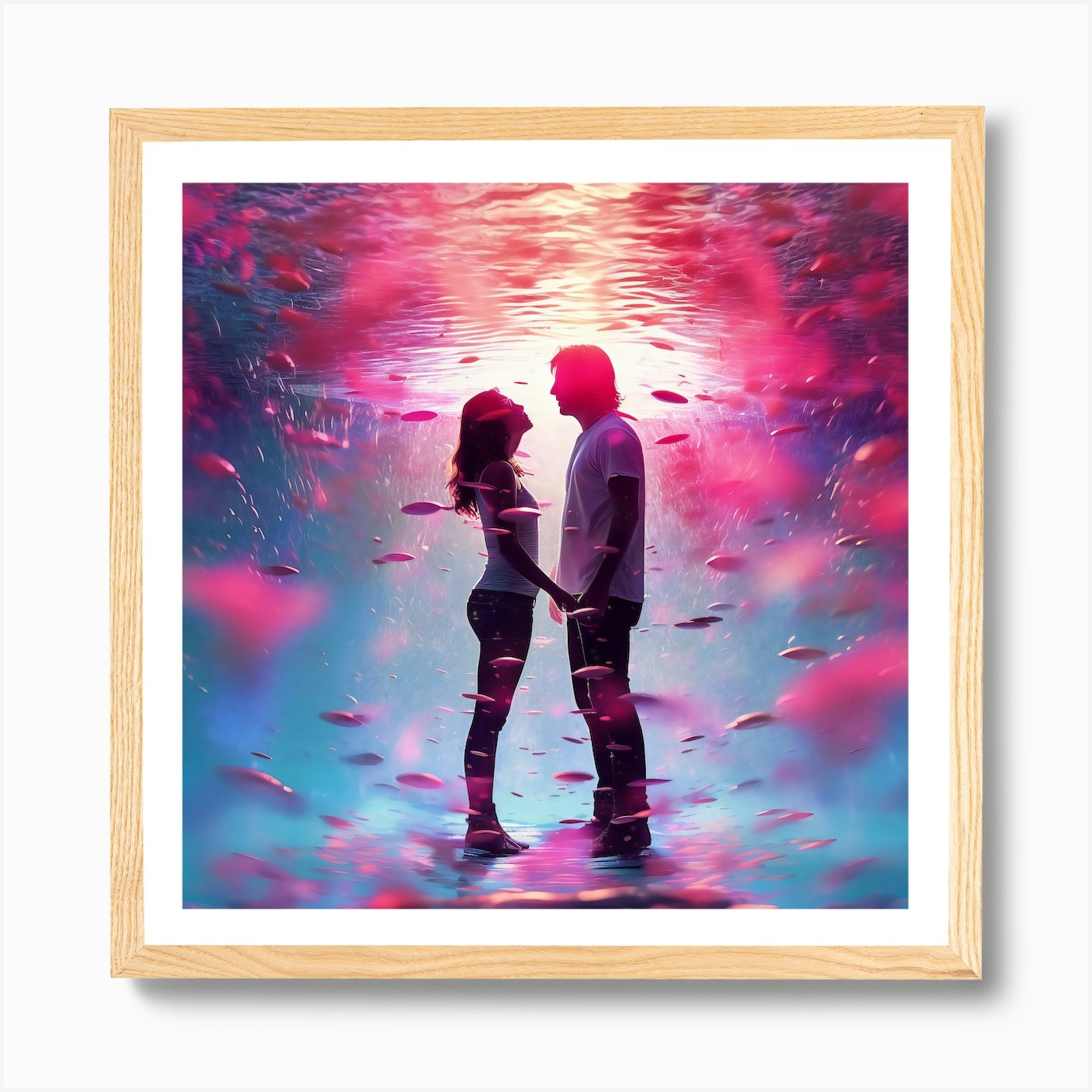The image features a framed piece of art hanging against a white wall. The simple, light-colored wooden frame surrounds a picture with a white border matting. The artwork itself appears to be an intricate composite photograph with a surreal, underwater theme. At the center, there is a young couple facing one another, their profiles highlighted. The woman, positioned on the left, is gazing up at the slightly taller man on the right as she stands a bit on tiptoe to hold his left hand with her right. Both are dressed in white t-shirts and dark jeans, with the woman's t-shirt being sleeveless. Surrounding them are vibrant hues of blue, accompanied by pink and red elements that resemble floating flower petals or bubbles and fish shapes, creating a dreamlike aquatic environment. A bright light or sunburst effect in the background enhances the ethereal quality of the scene, also producing hints of yellow and orange at the top, suggesting an illumination akin to sunlight filtering through water.